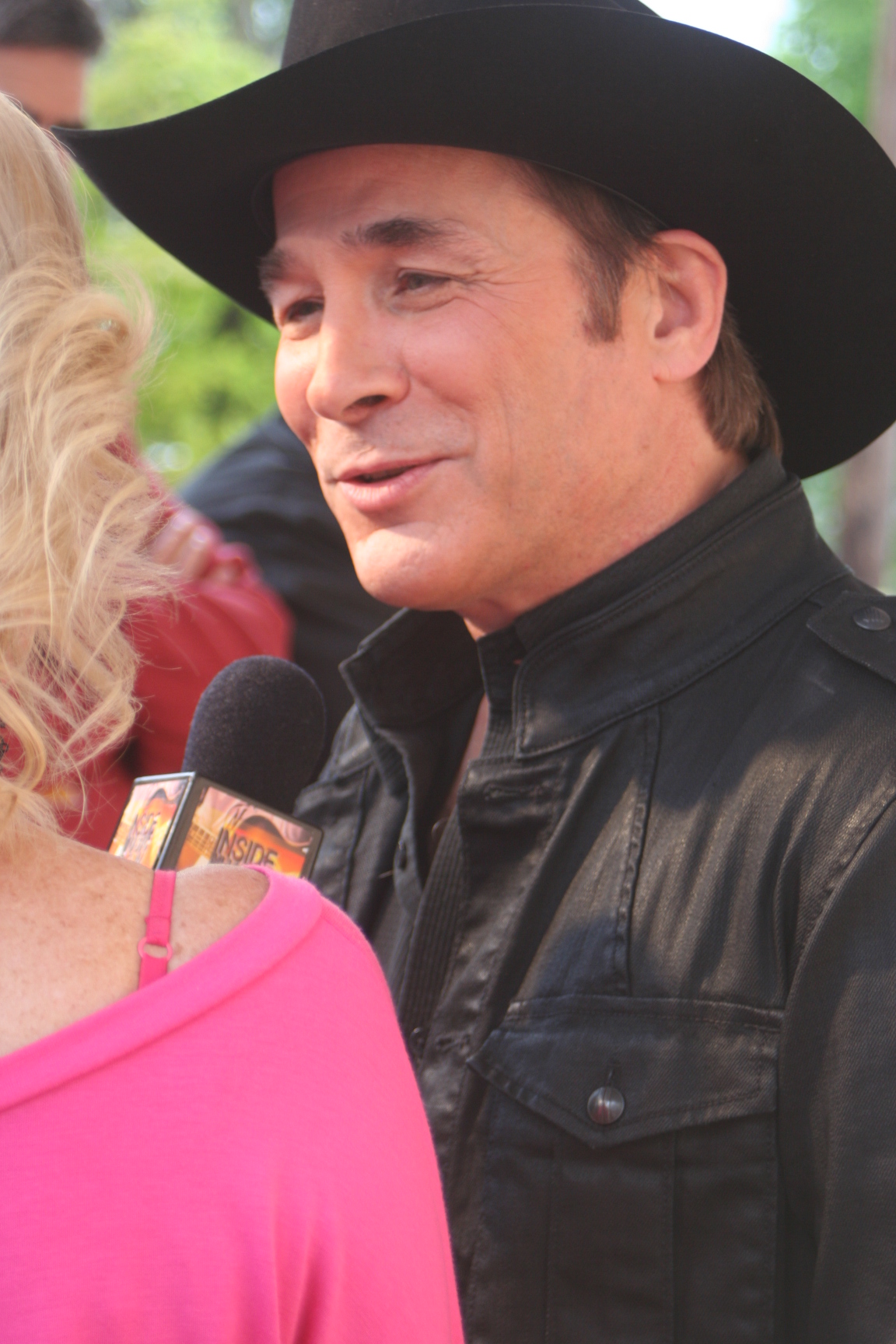In this outdoor image, country music star Clint Black takes center stage, dressed in a black leather jacket paired with a black cowboy hat, and sporting short brown hair. He is engaged in a conversation, smiling and addressing a woman to his left, who is holding up a microphone. The woman, captured from behind, wears a bright pink off-the-shoulder blouse with visible pink bra straps and has blonde, curly hair combed back. The microphone bears the partial inscription "inside," suggesting it could be from "Inside Edition." The background is blurry but hints at other people, including one in red and another in black, as well as a bit of greenery, indicating the scene is set outdoors.